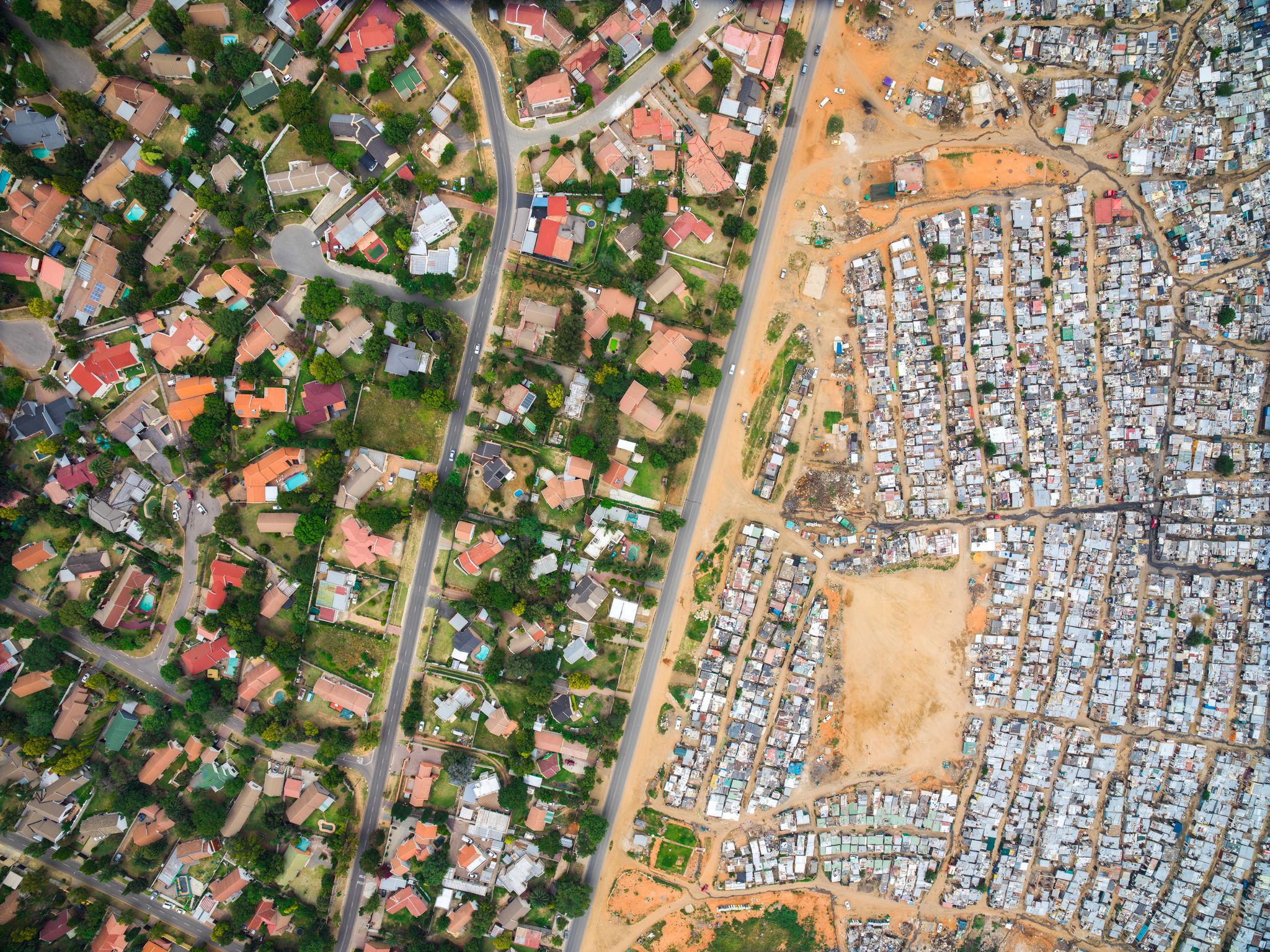This aerial image captures a striking contrast within a residential area, divided distinctly by a central roadway running diagonally through the scene. On the left, a lush, prosperous suburban neighborhood is characterized by larger, well-maintained homes, vibrant green lawns, and the presence of pools in some backyards. The streets here are in good condition, surrounded by numerous trees and greenery, suggesting an area that flourishes. Additionally, the terracotta roofs indicate it might be located in Southern California.

In stark contrast, the right side of the image reveals a densely packed urban environment with small, closely spaced homes, possibly shacks or motorhomes, in a desert-like landscape with little to no greenery. The buildings are primarily a uniform gray, with barren, brown lots interspersed among them, indicating a less prosperous and more impoverished setting. This juxtaposition of wealth and poverty, greenery and desert, creates a powerful visual divide within the same town, captured vividly from above.